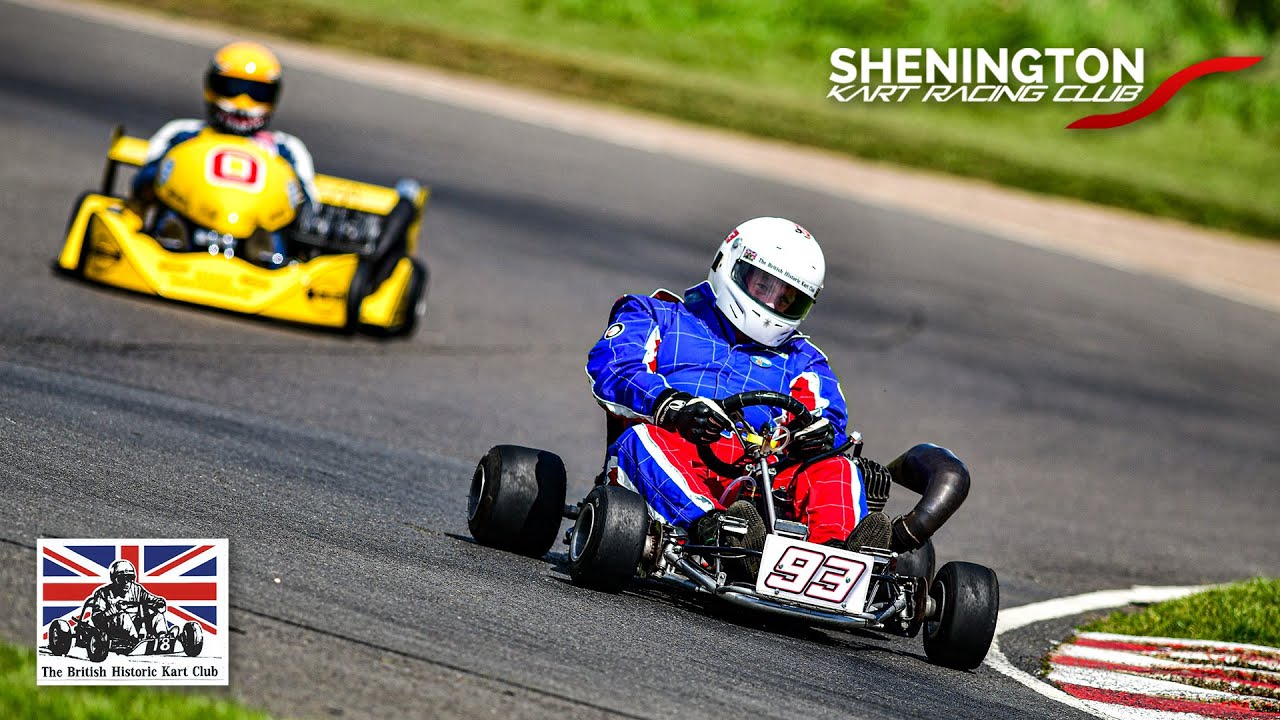This image is an advertisement for the Shennington Kart Racing Club, prominently displayed in white capital letters in the upper right corner with a small red ribbon nearby. The scene captures an outdoor go-kart race on a black asphalt track. Two racers are visible: the lead driver wears a white helmet and sports a blue and red outfit while driving a black go-kart marked with the white number 93; closely trailing is a racer in a yellow and black go-kart, distinguished by a yellow helmet. The lower left corner features a small square containing the British flag and a black-and-white drawing of a go-kart driver, labeled "British Historic Kart Club." Green grass is visible in the background, adding a vibrant contrast to the racing action.